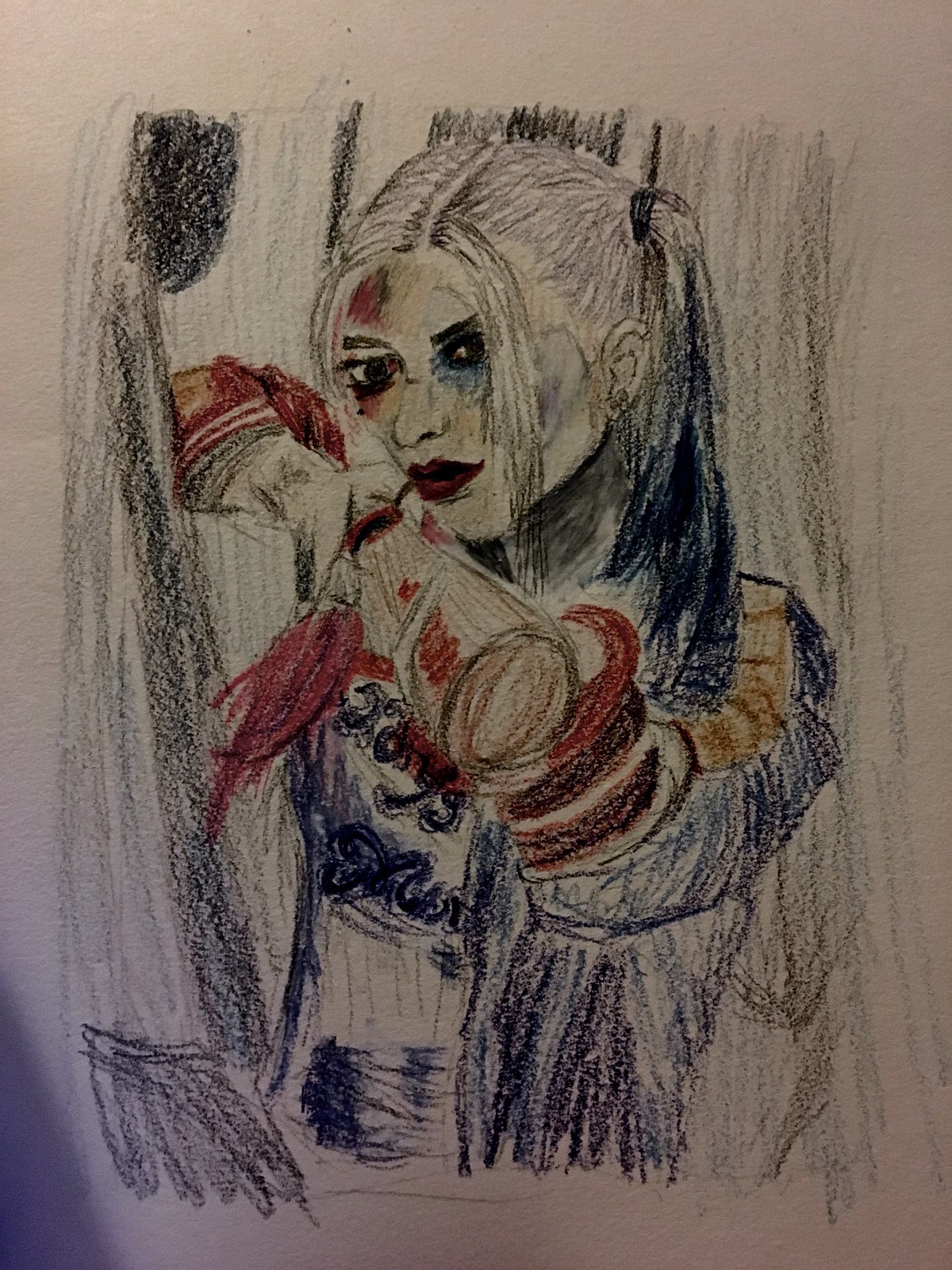This detailed colored pencil drawing captures the iconic character Harley Quinn from Suicide Squad. The artwork shows Harley facing the artist with a bold expression. She wears her signature blue and red jacket over a white shirt with indistinct blue text. Her left pigtail is dyed red and her right pigtail is blue, with the top of her hair remaining white. Her makeup is striking, featuring a predominantly white face with a blue right eye, a red left eye, deep red lips, and smudged mascara. The drawing includes realistic bruises and blood splatters, emphasizing the character's chaotic nature. Her left hand is raised as if pushing something away. The background is dark and shadowed, enhancing the vibrant colors of her outfit and adding depth to the piece. The drawing utilizes a mix of reds, blues, blacks, and subtle body details, such as blood on her arm, making it a compelling and vivid depiction of Harley Quinn.